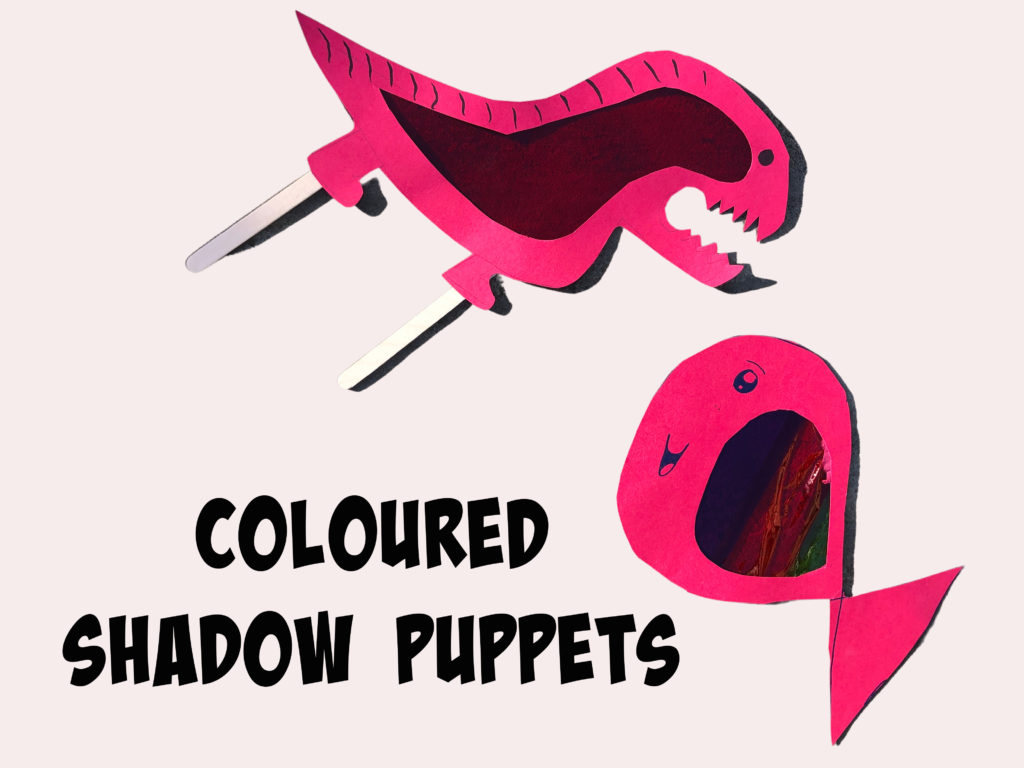The image depicts two bright pink shadow puppets against a white backdrop, with black all-caps text in the bottom left corner stating "COLOURED SHADOW PUPPETS." The first puppet resembles a creature with a circular orientation and dotted eyes, its neckline suggested by a triangular shape. The second puppet appears more intricate, resembling a bird-like dinosaur with an open mouth showcasing jagged teeth. This puppet stands on two posts, giving the impression it could be placed in the ground or another setting. Both puppets are primarily pink, with additional maroon coloring inside the mouth of the fish-like figure and the more intricate puppet.